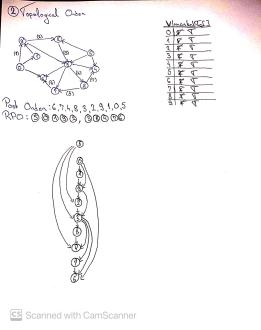This image showcases a scanned white piece of paper featuring varied elements, captured using CamScanner as indicated by the "CS" icon encased in a square on the bottom left. The paper is shadowed in both the upper left and right corners. 

On the upper right-hand side, there is a detailed list; although the specific words are illegible, it includes a column with numbers on the left and assorted symbols on the right, structured under a header separated by horizontal lines and aligned with a vertical line.

The left section of the paper has a "2" within a circle followed by an unclear word, beneath which lies a seven-sided diagram, resembling an incomplete octagon. Each of its vertices has lines extending towards the center, forming another set of segments converging at a central circle. Each vertex point contains small circles with minute numbers inside, and one of the triangles has an additional small circle at its center.

Below this is a list, commencing with an illegible word followed by several numbers, succeeded by another word and a second group of circled numbers. 

Further down, the paper displays another diagram – a vertical straight line featuring sequentially placed circles with numbers inside, interconnected by arrows, leading to an additional top circle with arrows branching out to the inferior circles. Adjacent to this diagram is an empty white space on the paper.